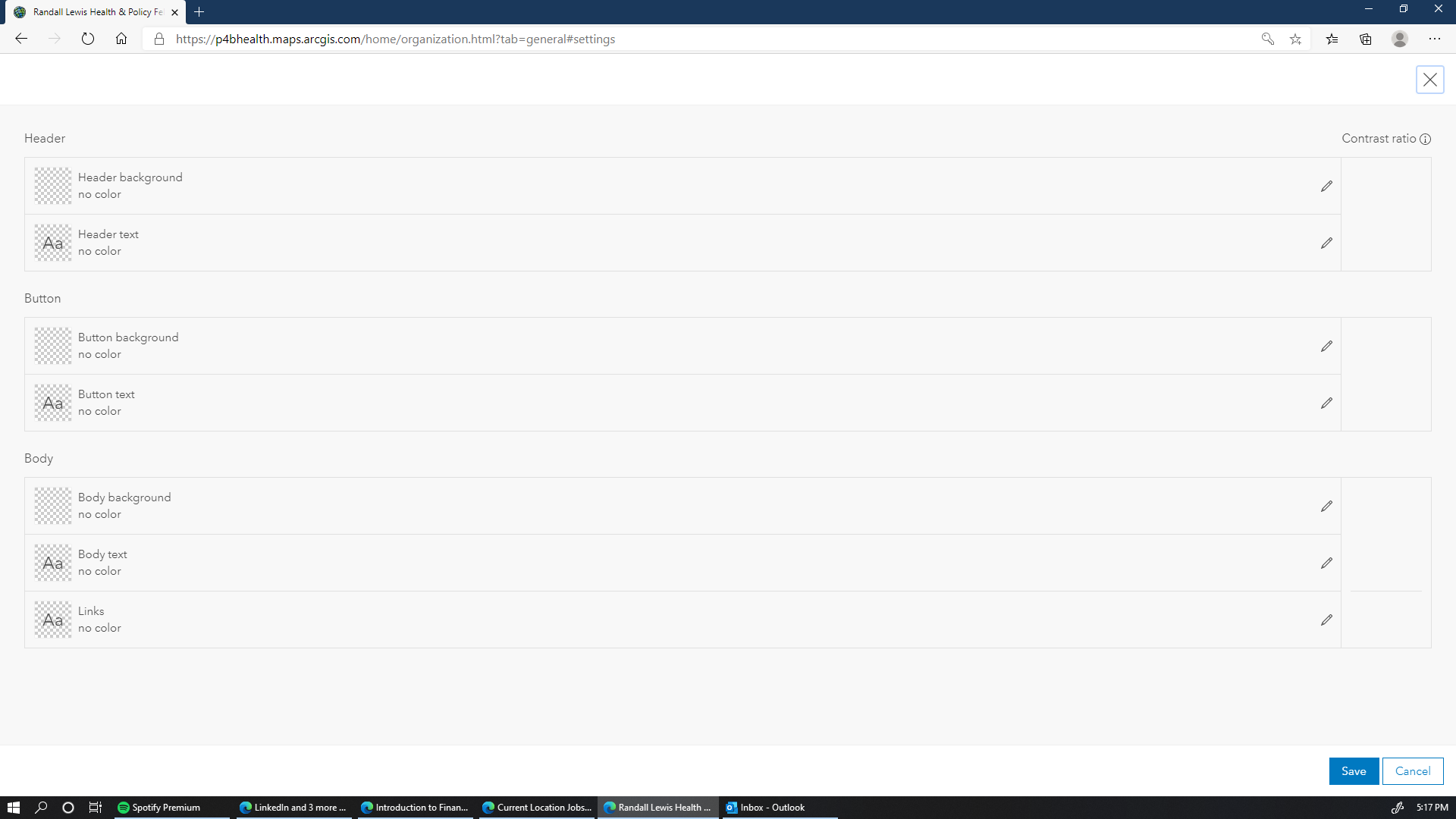This screenshot captures a computer screen displaying a specific webpage hosted at http://p4bhealth.maps.arkis.com. The image repeatedly emphasizes the web address http://p4bhealth.maps.arkis.com in its description, suggesting it's crucial to the context. The webpage likely relates to health-related maps provided by the Arkis platform, tailored for P4B Health's audience. The overall layout, visual elements, or specific data on the site are not detailed in the voice description, but the repeated focus on the URL underscores its importance to the content depicted.